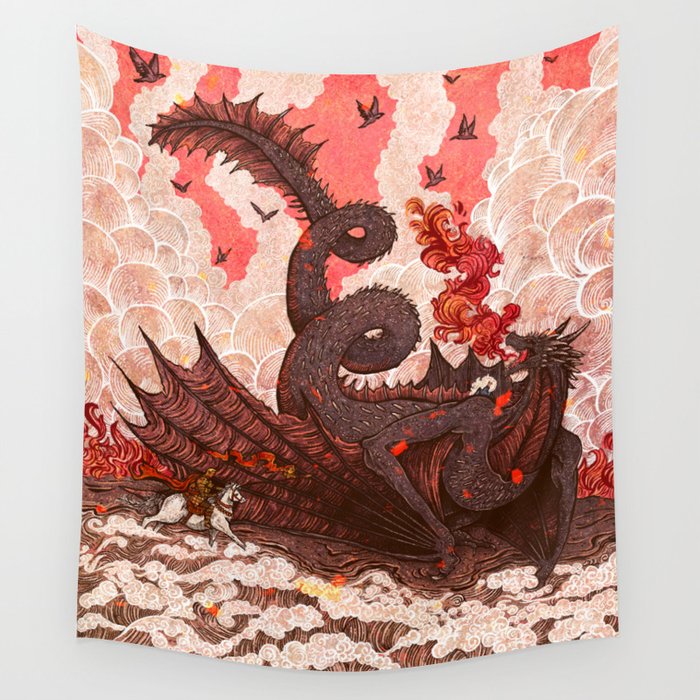The artwork is a detailed tapestry in the form of a banner hanging on a gray wall. Dominated by shades of pink, red, and black, the central figure is a massive black dragon with dark red wings and fins on the back of its tail. Spikes cover its body, leading up to its head, which is adorned with two horns. The dragon is depicted in an intense moment, blowing flames into the sky, suggesting it has just scorched the ground beneath. A tumultuous red sky forms the backdrop, with white clouds billowing from the fire raging on the ground. Birds are seen fleeing the scene, adding to the chaos. In the foreground, a small figure of a man in yellow armor rides a white horse, seemingly charging at the dragon with a long spear. The contrast in size emphasizes the dragon's immense presence compared to the man and his steed. The bottom of the tapestry features shades of brown, further grounding the fiery and chaotic scene above.